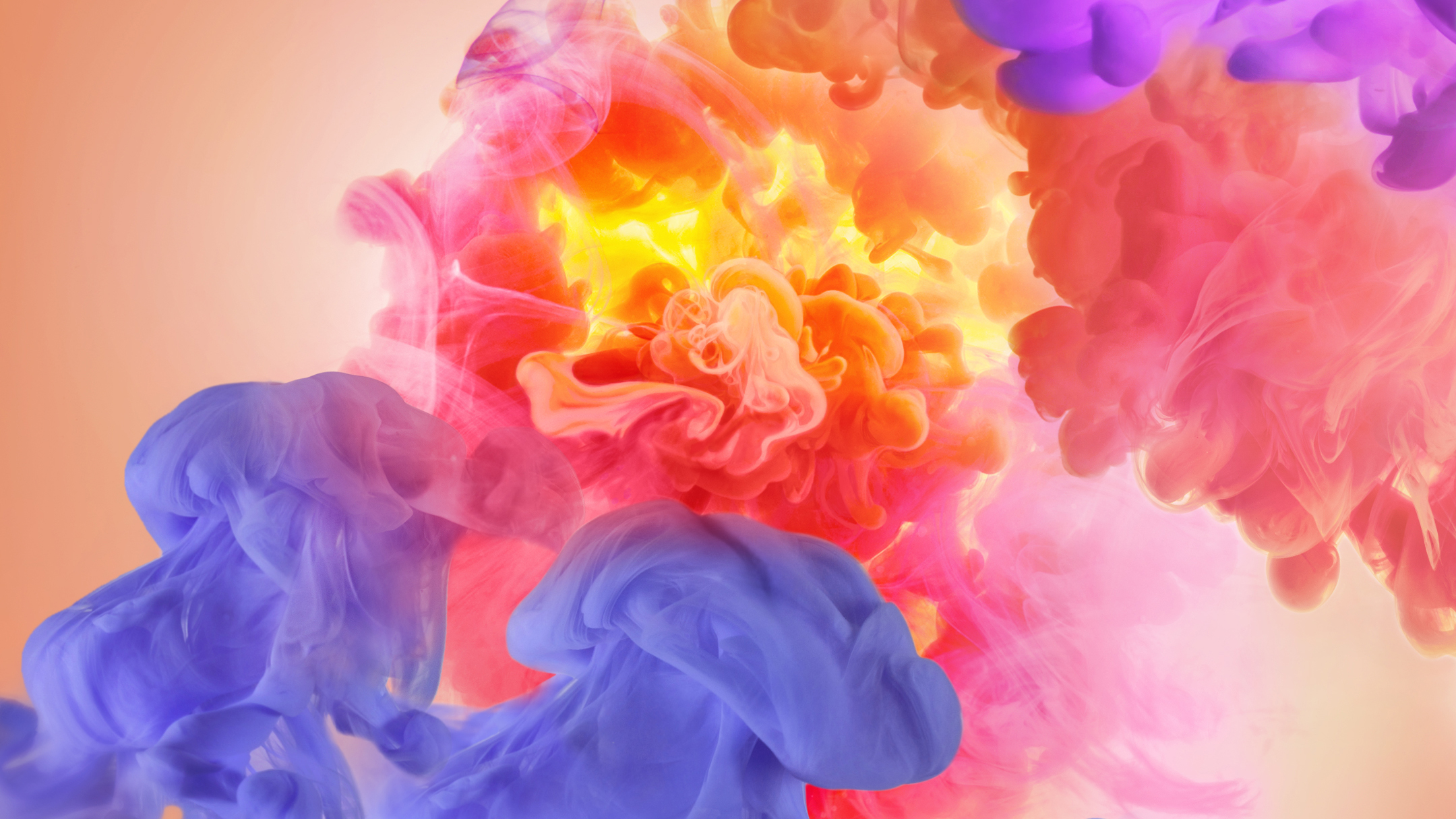This is an intricate piece of digital abstract art featuring a vibrant, smoke-like composition reminiscent of tie-dye patterns. The background radiates a soft salmon pink, gradually lightening towards the middle into a pinkish white shade. The centerpiece is dominated by a billowing formation of bright orange and red hues, resembling a flowery bloom with striking yellow highlights at its core. Surrounding this central motif are luminous clouds of smoke, with vivid pinks, oranges, and touches of white. Extending from the bottom, rich royal blue plumes sweep upwards, transitioning into shades of purple in the upper right and blending with additional red and pink trails. Particularly notable are two large, jellyfish-shaped billows in dark blue situated in the lower left, contrasting with the purplish smoke tendrils in the top right. This visually captivating canvas showcases a complex interplay of color and form, conveying a sense of dynamic movement.